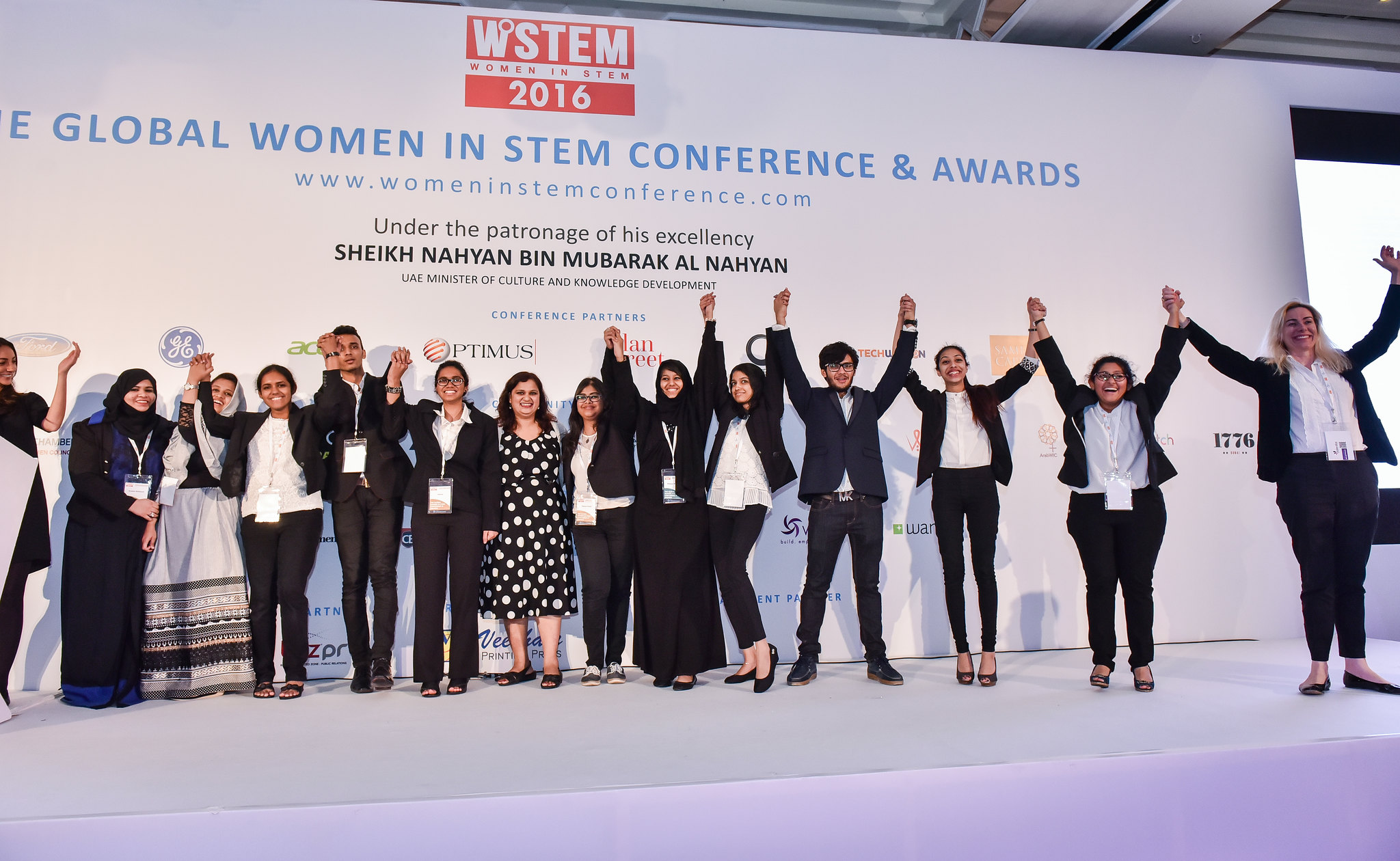A group of attendees, both men and women, are standing on a stage with their hands raised in the air, celebrating at the Global Women in STEM Conference and Awards 2016. The stage and background are primarily white with a large banner featuring the event details. At the top of the banner, in red text against the white background, it reads "WSTEM," which stands for Women in STEM (Science, Technology, Engineering, and Mathematics). Below that, the year "2016" is displayed in red. Further down in blue letters, it says "Global Women in STEM Conference and Awards," followed by the website "www.womeninstemconference.com." Below that, in black lettering, the banner states, "Under the patronage of His Excellency Sheikh Nahyan bin Mubarak Al Nahyan, UAE Minister of Culture and Knowledge Development." Various partner logos are also visible on the banner. The attendees are dressed in formal attire, including long dresses, pantsuits, and jackets, with some men wearing jeans. The scene is one of celebration and unity, with the primary colors in the image being light lavender, blue, red, and black.